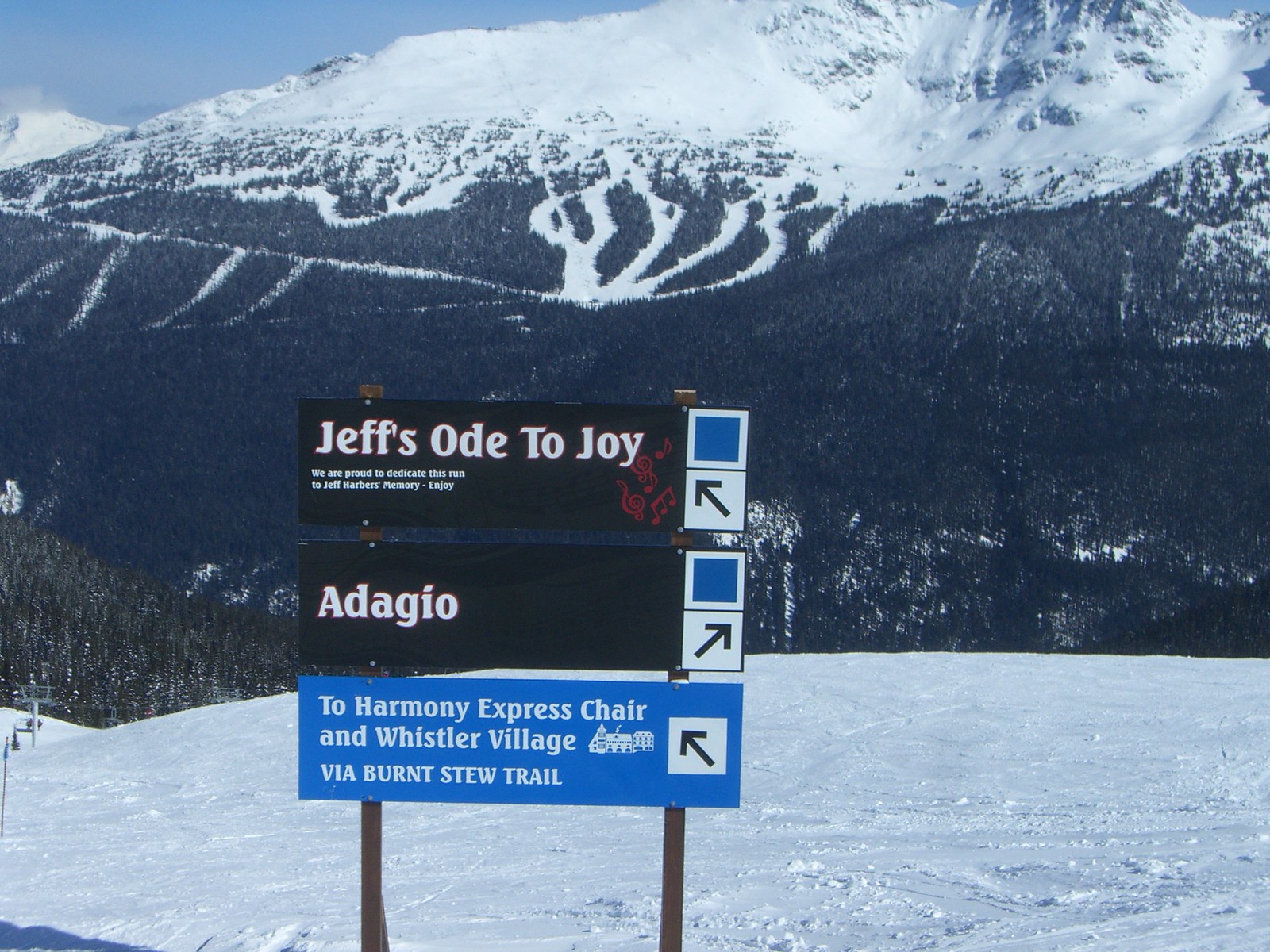The image depicts a scenic snowy mountain with a clear blue sky, captured during the daytime. The majestic mountain, adorned with patches of snow, rises in the background, while clusters of trees inhabit the lower slopes. The ground in the foreground is blanketed with snow, where a wooden stand supports three signs.

The top sign, with a black background, reads "Jeff's Ode to Joy" in white letters, accompanied by an arrow pointing left and a red musical note logo, and a dedication to Jeff Harbour's memory and joy. Below it, another black-background sign reads "Adagio," featuring an arrow pointing right and similar logos, including blue and white squares. The bottom sign has a blue background and directs visitors to "Harmony Express Chair and Whistler Village via Burnt Stew Trail," with an arrow pointing left and corresponding logos. This arrangement underscores a tribute to Jeff Harbour, guiding visitors through the snowy landscape towards different destinations.